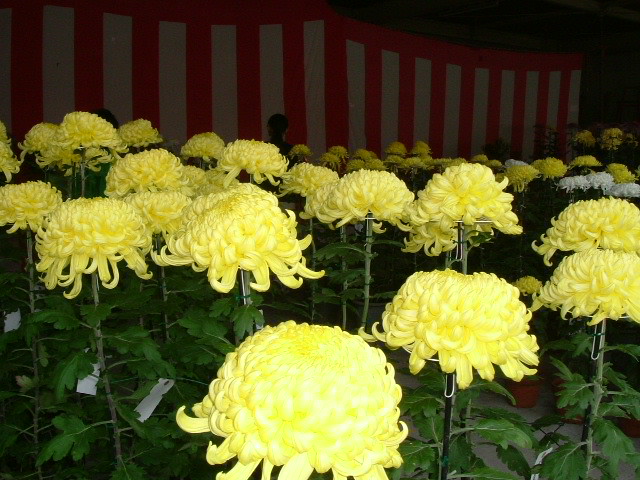A close-up of vibrant yellow flowers with curly petals, each radiating from a round central disc, stands prominently against a striking background of red and white stripes. The lush green stalks support an impressive array of blooms—counting over twenty in this frame alone—with additional flowers trailing into the background. Among these sunlit blossoms, darker yellow variations can be observed, interspersed with white versions on the right side. In the distant background, a woman with a brown ponytail adds a human element to the scene, subtly contrasting with the botanical splendor in the foreground.